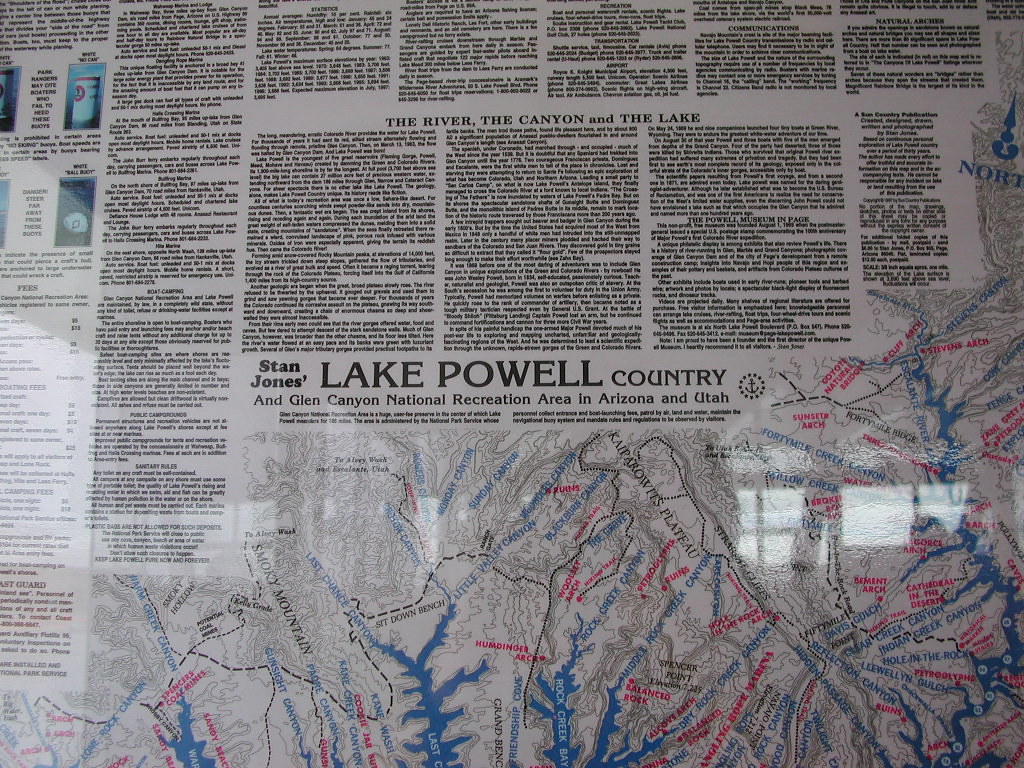This photo captures a detailed wall hanging or framed print titled "Stan Jones' Lake Powell Country and Glen Canyon National Recreation Area in Arizona and Utah." It is encased in either plexiglass or a glass frame, as indicated by the visible reflections of windows opposite the display. The central section is dominated by a map that stretches diagonally from the top right to the bottom left, illustrating routes and locations in vivid blue, red, and gray colors. Above the map, the wall hanging features a heading, split into prominent titles, "The River, The Canyon, and The Lake," and the larger "Lake Powell Country Stan Jones," accompanied by an anchor logo. Small text underneath provides additional context, although it is difficult to read in its entirety due to the detailed and fine print. To the left side of the map, two columns contain further explanatory text, contributing to the overall informative nature of the display. The reflections on the glass suggest it is hung on a large wall, emphasizing its expansive and detailed presentation.